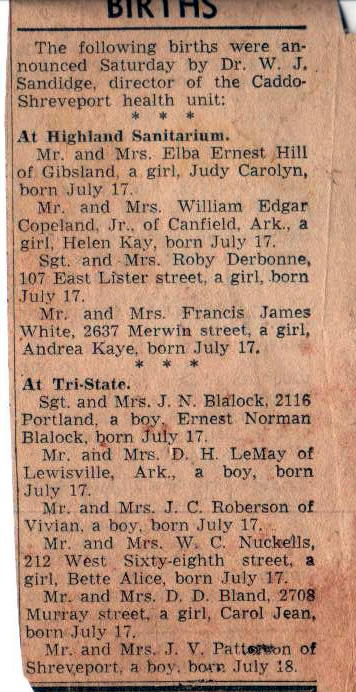The image is a worn and old-fashioned newspaper clipping listing births, under the heading "BIRTHS" in bold black capital letters with a black line underneath. It details the births announced on a Saturday by Dr. W.J. Sandage, Director of the Caddo Shreveport Health Unit, with entries divided by asterisks. At Highland Sanitarium, Mr. and Mrs. Elba Ernest Hill of Gibsland welcomed a girl, Judy Caroline, on July 17th. Mr. and Mrs. William Edgar Copeland, Jr. of Canfield, Arkansas also celebrated the birth of a girl, Helen Kay, on the same date. Sergeant and Mrs. Roby Durbin of 107 East Lister Street had a girl on July 17th, while Mr. and Mrs. Francis James White of 2637 Merwin Street announced the birth of their girl, Andrea Kay, on July 17th as well. At Tri-State, Sergeant and Mrs. J.N. Blaylock of 2116 Portland had a boy, Ernest Norman Blaylock, on July 17th. Additionally, Mr. and Mrs. D.H. LeMay of Louisville, Arkansas, Mr. and Mrs. J.C. Robertson of Vivian, and Mr. and Mrs. W.C. Knuckles of 212 West 68th Street each celebrated boys born on July 17th, with Betty Alice born to Mr. and Mrs. Knuckles and Carol Jean born to Mr. and Mrs. D.D. Bland of 2708 Murray Street. Lastly, Mr. and Mrs. J.V. Patterson of Shreveport announced the birth of a boy on July 18th. The condition of the clipping suggests it dates back to the 70s or 80s.